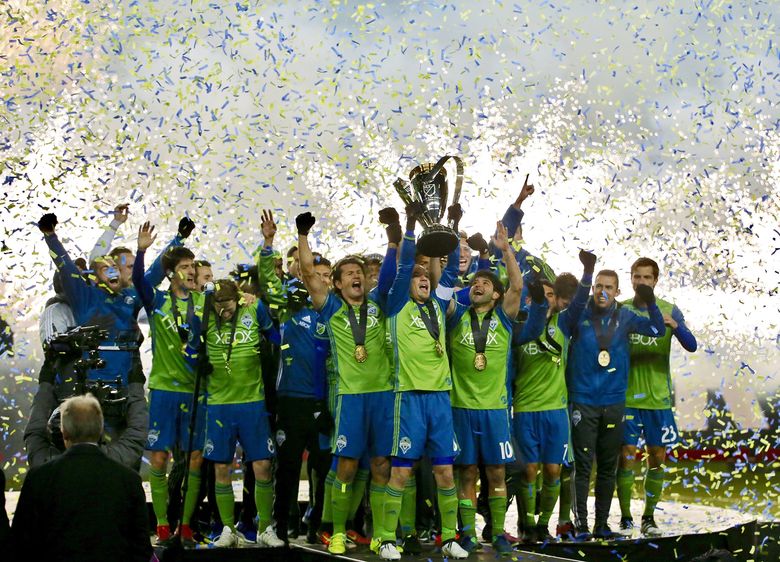In this vibrant landscape-oriented image, a jubilant soccer team is celebrating their championship victory on a black platform. The players, gathered closely together with their arms raised in triumph, are adorned in distinctive green jerseys with blue sleeves, complemented by blue shorts featuring green stripes along the sides. Their ensemble is completed with bright green socks covering shin guards, and variously colored shoes - some white, red, and orange. Each player proudly wears a medal with a gold emblem, suspended from blue or black ribbons around their necks. The jerseys prominently display "Xbox" as the team sponsor. Visible jersey numbers include 7, 8, 6, 10, and 23, while the shorts also bear white numbers on the left and a green and white logo on the right. Central to the celebration, one player holds aloft a large gold trophy. The air is filled with an explosion of blue, green, and white confetti, white fireworks, and translucent fog, enhancing the festive atmosphere. In the background, people are capturing the moment with cameras, including a man in a suit and other individuals dressed differently from the team.